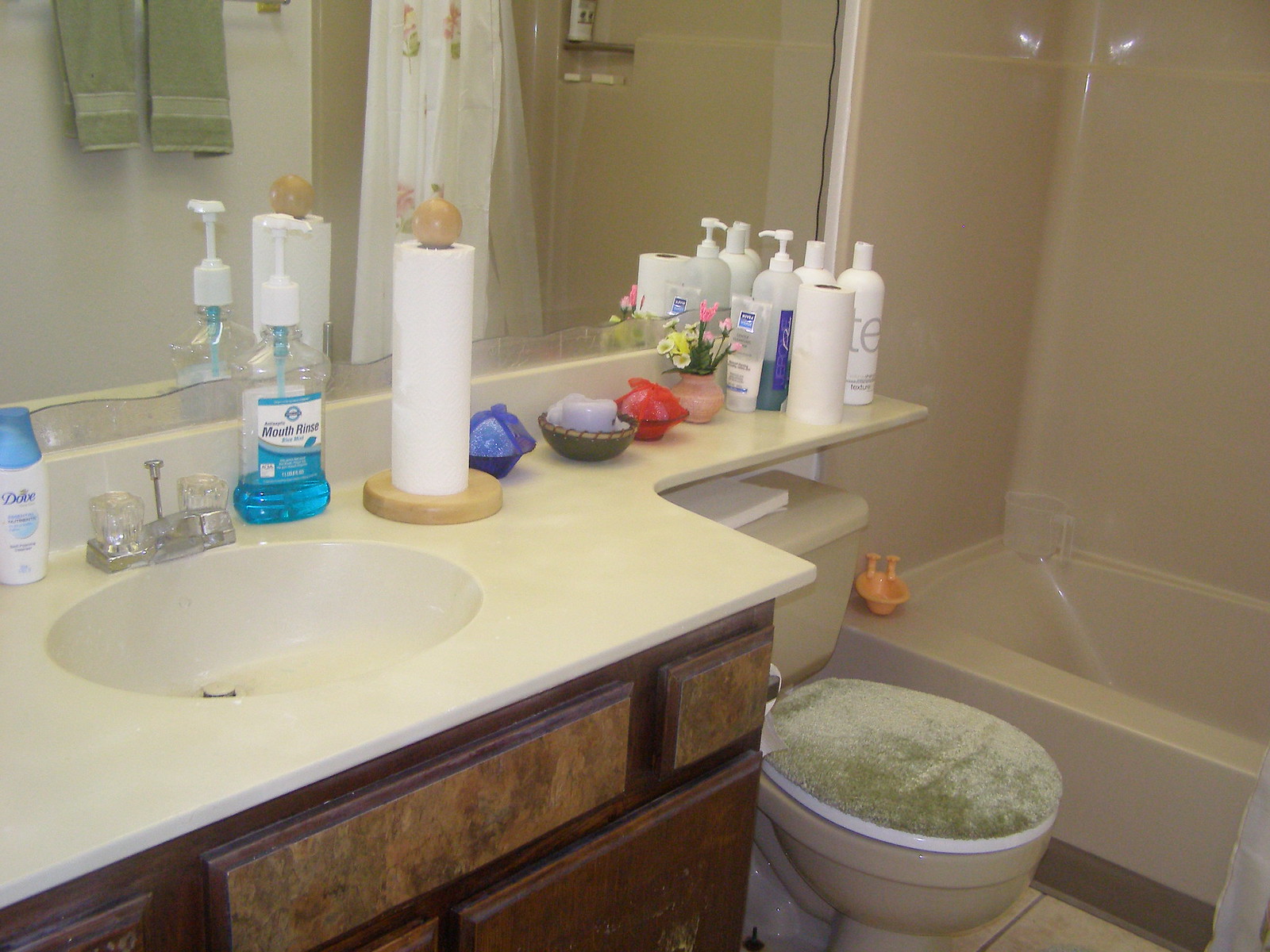This image showcases a cozy, well-maintained bathroom with a mix of dated and contemporary elements. At the heart of the space is a wooden cabinet beneath the sink, which displays signs of wear and a dingy, lived-in appearance. In contrast, the toilet gleams with newness, featuring a pristine beige toilet seat cover and matching toilet body. Adjacent to it is a shower surround and a large beige bathtub, both appearing brand new. A small yellow toy, likely a child's, sits on the left side of the tub, adding a touch of personality to the bath area. 

The bathroom floor looks freshly refurbished as well, though only a single tile near the toilet is visible. The sink, an elegant lighter beige oval integrated unit, extends above the toilet, maximizing the counter space. This extended counter holds several personal care items, including a bottle of mouth rinse and a Dove product, among other toiletries. 

Adorning the countertop are a few decorative knickknacks, such as a pink vase with flowers and a paper towel roll situated centrally. The expansive, spotless mirror behind the sink reflects various elements of the bathroom: two sage-green hand towels, a white shower curtain, and a cubby within the shower holding a single bottle. Overall, the room balances well-used features with fresh upgrades, creating a functional and welcoming atmosphere.